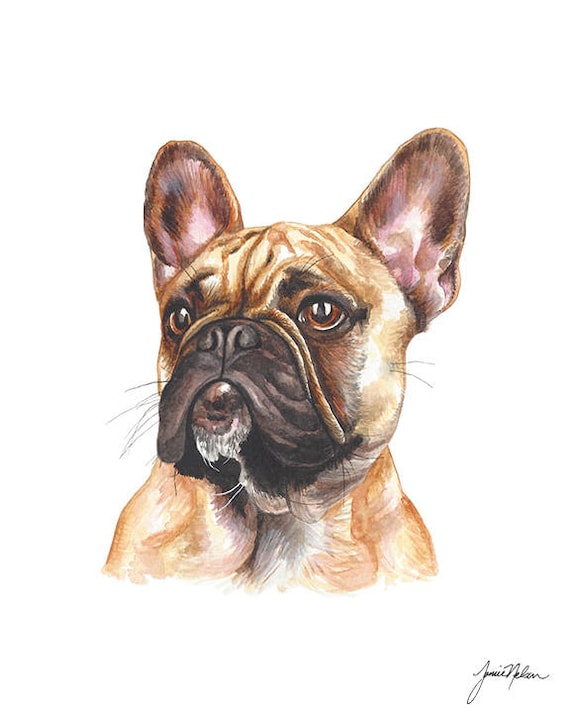The image features a detailed and realistic portrait of a pug dog, set against a white background. The artwork, which appears to be created using a blend of watercolor and pencil techniques, captures the pug from the shoulders up. The pug's coat is primarily a light brown caramel color, with a touch of white under its chin and darker areas beneath its wrinkles. The dog's face is distinctly flat with plentiful wrinkles, a black snout, and a black nose. Its large, bright brown eyes are spaced widely apart, adding to its endearing expression. The pug's ears stand upright, featuring dark edges and pink interiors. A signature at the bottom of the portrait, which might read "Jamie Nellen" or "Janice Nelson" in cursive, identifies the artist. The pug is positioned to look towards the left side of the image, showcasing both its charming facial features and its slightly wrinkled forehead. The combination of watercolor and pencil gives the portrait a lifelike texture and depth, making it a captivating representation of the pug.